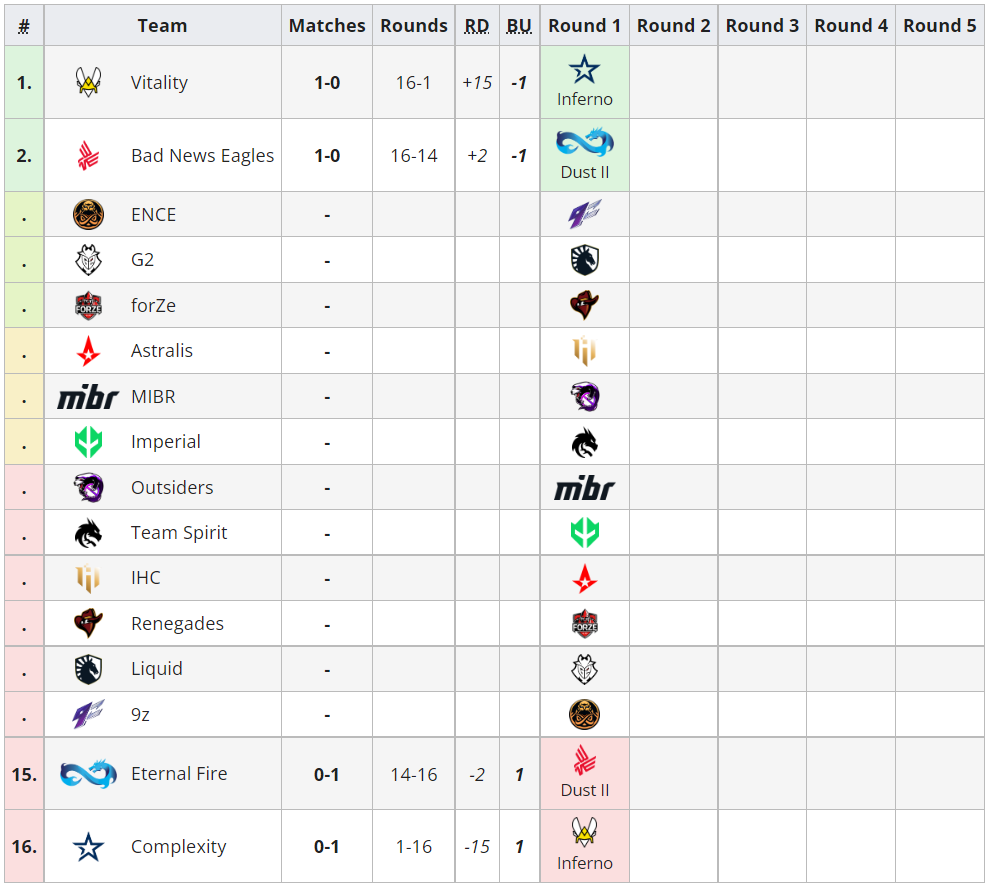The image displays a screenshot of a detailed spreadsheet designed to track the progress of a tournament. The spreadsheet is organized with columns for team names, match results, and various rounds. Starting from the upper left-hand corner, the columns are labeled: "#", "Teams", "Matches", "Rounds", "RD", "BU", followed by "Round 1", "Round 2", "Round 3", "Round 4", and "Round 5". 

Each team name is listed in descending order down the first column, though only a few numbers are assigned. For instance, "#1" is assigned to "Vitality" and "#2" to "Bad News Eagles", but subsequent numbers are skipped, reappearing at #15 for "Eternal Fire" and #16 for "Complexity", which is marked with a star symbol.

The teams listed include: 
1. Vitality
2. Bad News Eagles
3. Ent
4. G2
5. 4ZE
6. Australis
7. MIBR
8. Imperial
9. Outsiders
10. Team Spirit
11. IHC
12. Renegades
13. Liquid
14. 9Z
15. Eternal Fire
16. Complexity

Currently, the spreadsheet is partially filled, with only Round 1 completed and rounds 2 to 5 remaining blank. Match results so far indicate scores such as "1-0" and "0-1", with some areas still awaiting information. The intricate layout suggests an organized approach to documenting and tracking the tournament's progression, reflecting the dynamic nature of the competition.